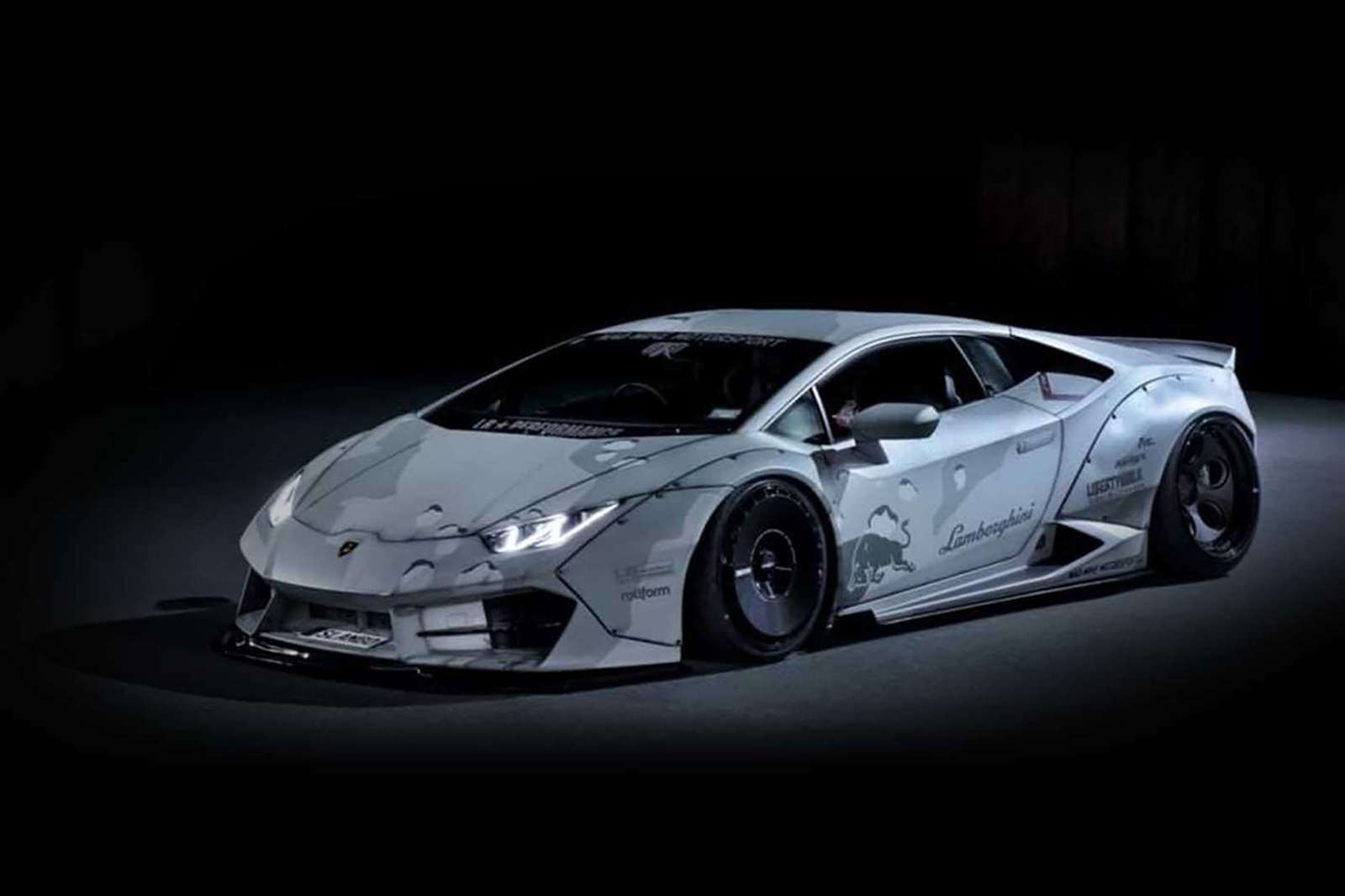This photograph depicts a sleek Lamborghini sports car, presented in a black and white format, emphasizing its luxurious and aerodynamic design. The car appears silver or gray, though the monochrome nature of the image makes precise color determination difficult. The photo showcases the left-hand side, including the driver's side door emblazoned with the word "Lamborghini" and featuring a gullwing design. The vehicle is positioned against a dark, black background, with a subtle circle of light beneath it highlighting the Lamborghini's graceful lines and curves. Notable features include its sloped rooftop, rear spoiler, large black rims with prominent tires, and a dynamic, riveted side design that resembles a camouflage print. The image captures the essence of the Lamborghini's high-end luxury, set on a dark gray floor with a dim spotlight accentuating its contours.